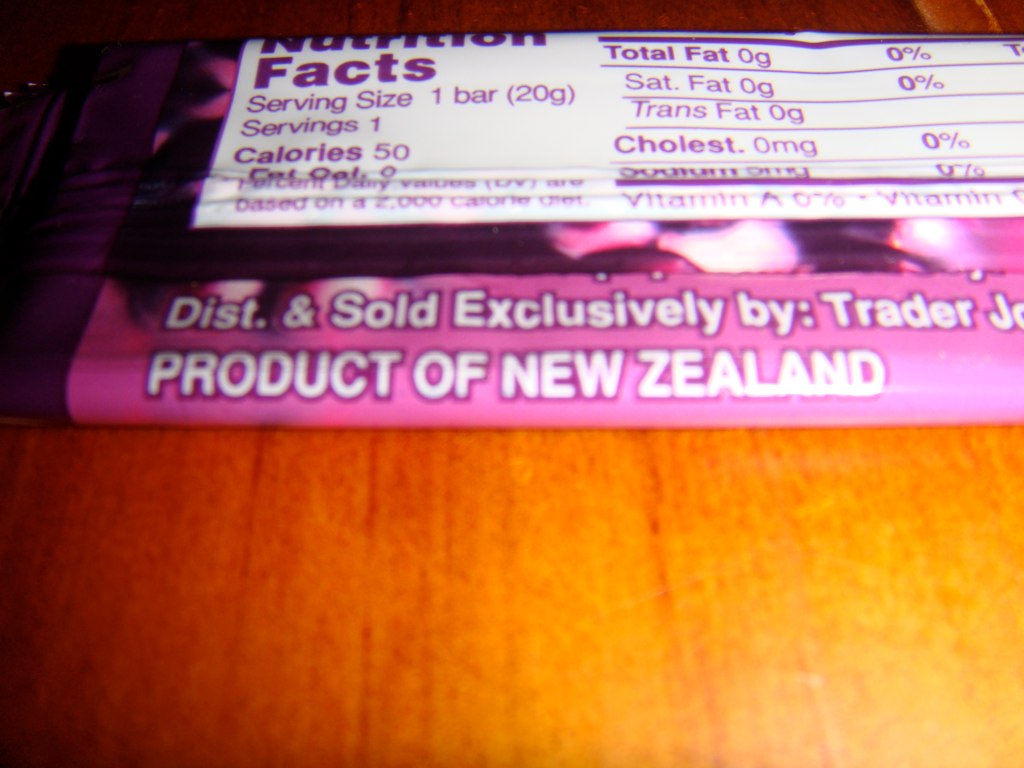The image features a product that appears to be a candy bar wrapped in pink and white packaging. The bottom of the wrapper has text in white letters that reads "D-I-S-T period" and mentions that the product is distributed and sold exclusively by Trader Joe's, although only the letter 'J' is visible because the rest of the label is cut off. In all capital letters, it states that the product is from New Zealand. Above this, there are nutritional facts written in purple text. It lists the serving size as one bar, with a calorie count of 50 per serving. The product contains no fat, trans fat, cholesterol, vitamin A, or sodium. The image is somewhat dark on the left side, but there appears to be a glimpse of chocolate peeking out, although it is not entirely clear. The item is placed on what looks like a wooden table.